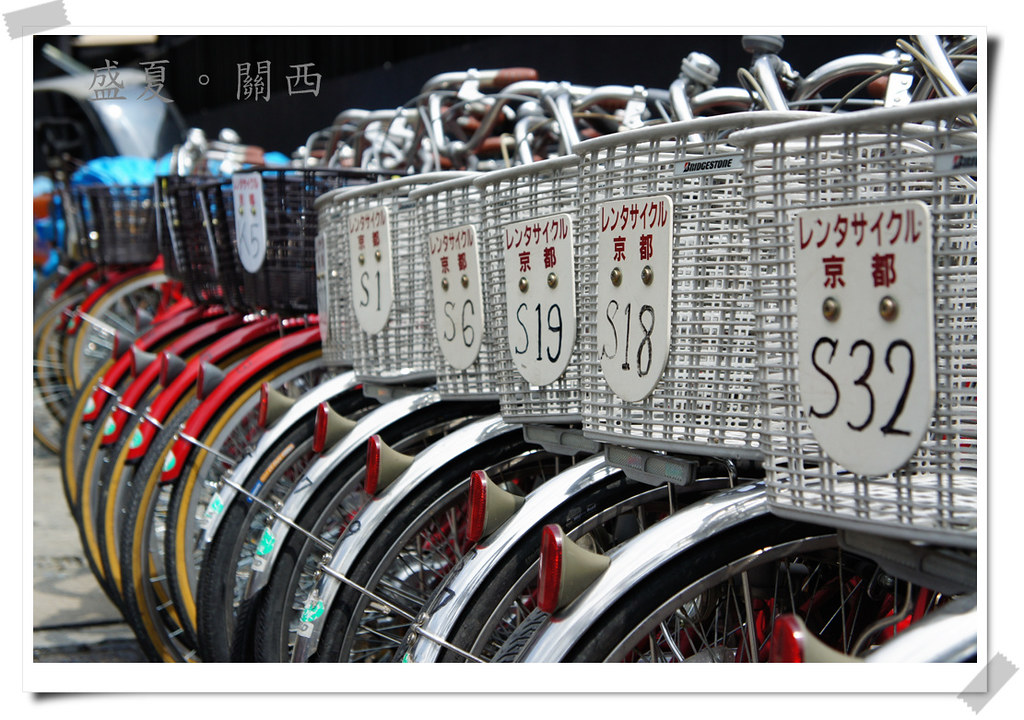The image depicts a tightly arranged display of bicycles, captured in an extreme close-up that highlights only the front wheels, fenders, baskets, and part of the handlebars. The bicycles are aligned side by side, with tires extending from the middle left to the bottom right of the frame. Half of the bicycles feature red fenders with black baskets, while the other half have silver fenders with matching silver or gray baskets. On each basket, there are white cards with Chinese writing and specific identifiers: S1, S6, S19, S18, and S32. The background shows additional bicycles, but their details are less distinct. The top of the image contains more Chinese text and symbols, which provide additional context to the scene. The intricate arrangement and diversity of the bicycles' features are accentuated by the contrasting colors of the fenders and baskets.